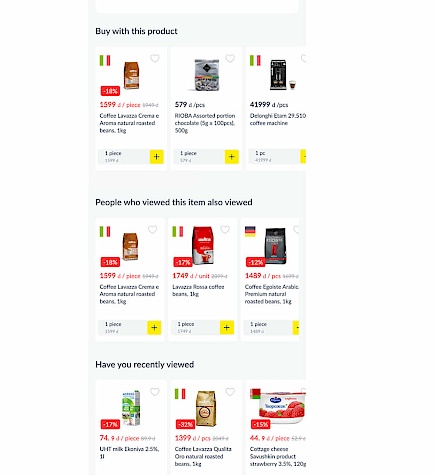This is a detailed description of a screenshot taken from a phone displaying a shopping page with various purchasable items, organized into three sections.

**Top Section: "Buy with this Product"**
- **Left:** A bag of coffee, presented with a price and a percentage reduction highlighted in a red box. There is an option to add the item to your cart by clicking on a yellow box with a plus sign.
- **Middle:** A silver bag of chocolates, depicted with an image of chocolates on the front. The price and quantity of pieces are mentioned. The item can be added to the cart via the yellow plus sign button.
- **Right:** A black and silver coffee machine, featuring a clear glass cup filled with coffee below it.

**Middle Section: "People Who Viewed This Item Also Viewed"**
- **Left:** The same bag of coffee as shown in the top section.
- **Middle:** A red and white bag of coffee with a 17% reduction.
- **Right:** A black bag of coffee with a label on the front, also reduced by 17%. Each of these items can be added to the cart using the yellow plus sign button.

**Final Section: "Have You Recently Viewed"**
- **Left:** A white box with green detailing on the front, offering 17% off.
- **Middle:** A gold bag of coffee, showing a 32% reduction.
- **Right:** A single-serving yogurt container, featuring strawberries on the front and marked down by 15%.

Each item in all three sections has the option to be added to the cart through a yellow box featuring a plus sign.